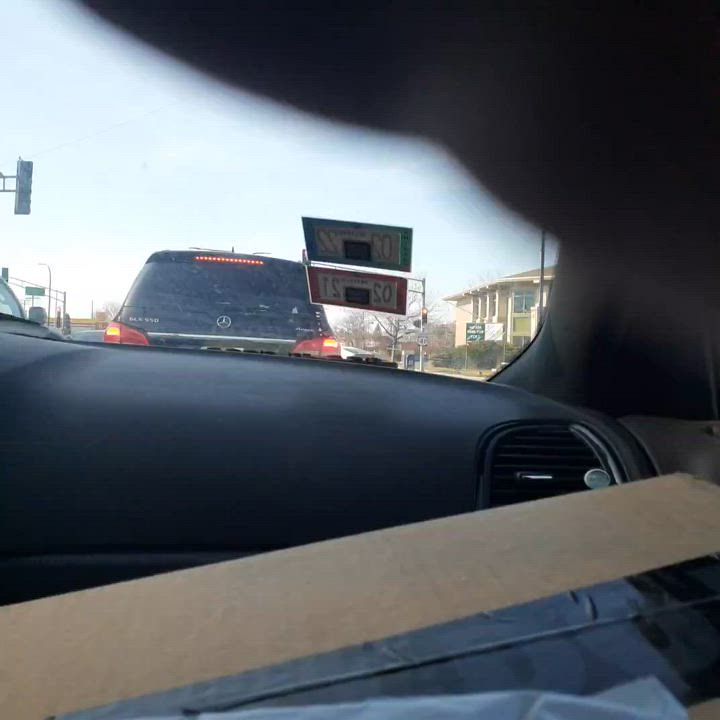The photograph captures a view from the front windshield of a car. The lower section of the image features a light blue hue, transitioning into a series of gray rectangles, indicative of reflections or dashboard elements. Prominently, a large gray rectangle stretches diagonally upward to the right across the frame, leading to the black dashboard of the car. On the right side of the dashboard, a vent is clearly visible. The upper right corner and almost to the left edge features a very blurred black area, possibly part of the car's interior.

Through the windshield, the rear of a black SUV is in clear view. To the right, there is a one-story tan building. Just at the left edge of the frame, a sign is hanging, though its details are not discernible. The sky above is a clear, vibrant blue, adding to the sense of a bright day.